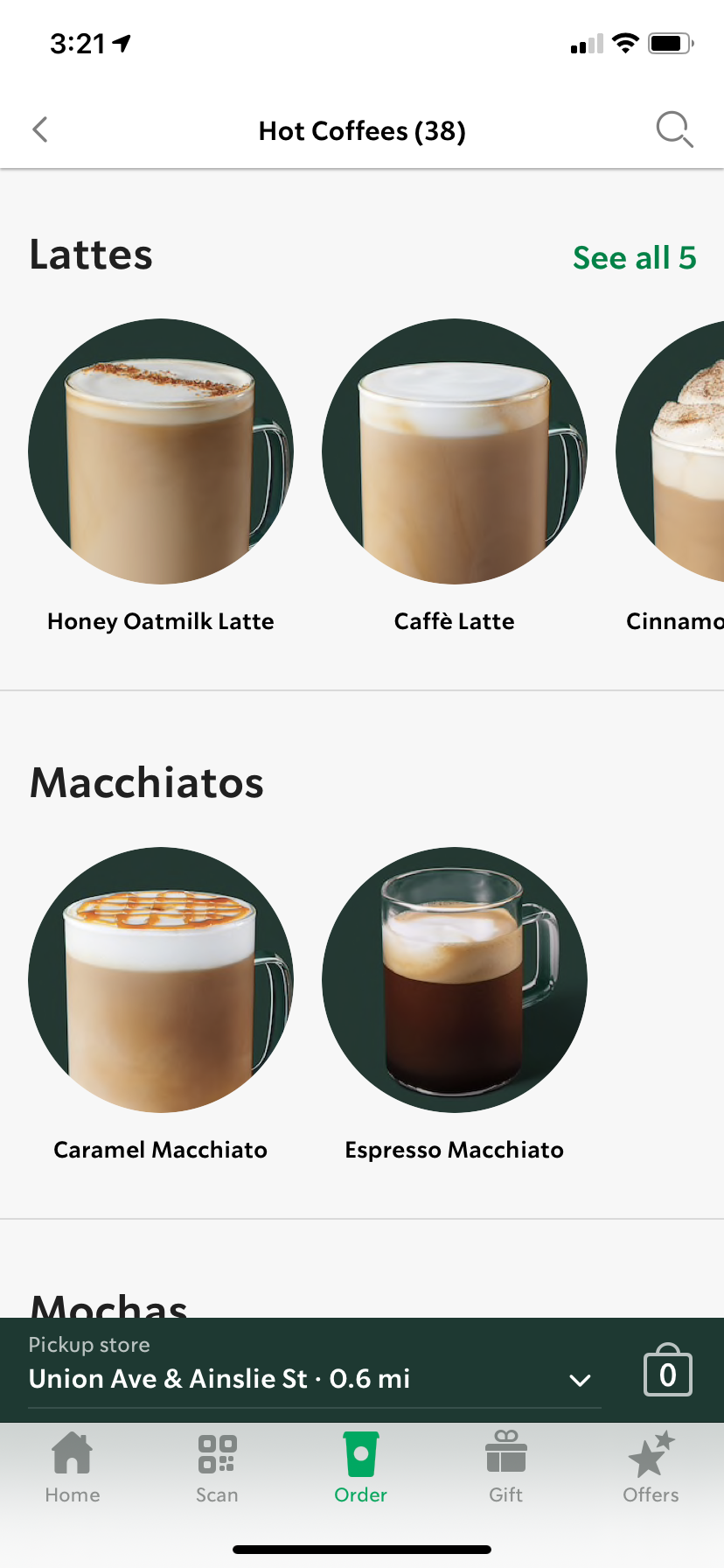This is a detailed vertical screenshot of a mobile app, likely for Starbucks. The interface displays a variety of elements with precision. 

In the top left corner, the text "321" appears accompanied by a location symbol. On the right side, indicators show the service strength at 2.4 bars, a WiFi symbol, and a battery icon that appears to be between 80% and 90% charged.

The focal point of the screenshot is the "Hot Coffees" section, which lists 38 options. A back button is located on the left, while a search icon is situated on the right. Below, images of different lattes are displayed, labeled with "CO5" in green. The visible lattes include a Honey Oat Milk Latte, a Coffee Latte, and a Cinnamon Latte, though the latter is partially cut off. 

The next section features "Macchiatos," displaying options such as Caramel Macchiato and Espresso Macchiato. Below this, there is a partially visible section for "Mochas."

Further down, a green background bar indicates a nearby store: "Union Avenue and Ainsley Street," located 0.6 miles away. A drop-down list allows the selection of a different store. An icon shows an empty cart with a "0" next to it.

The bottom navigation bar includes a "Home" button, a "Scan" button, and a highlighted "Order" button in green. Additionally, there are buttons for "Gift" and "Offers for Stores."